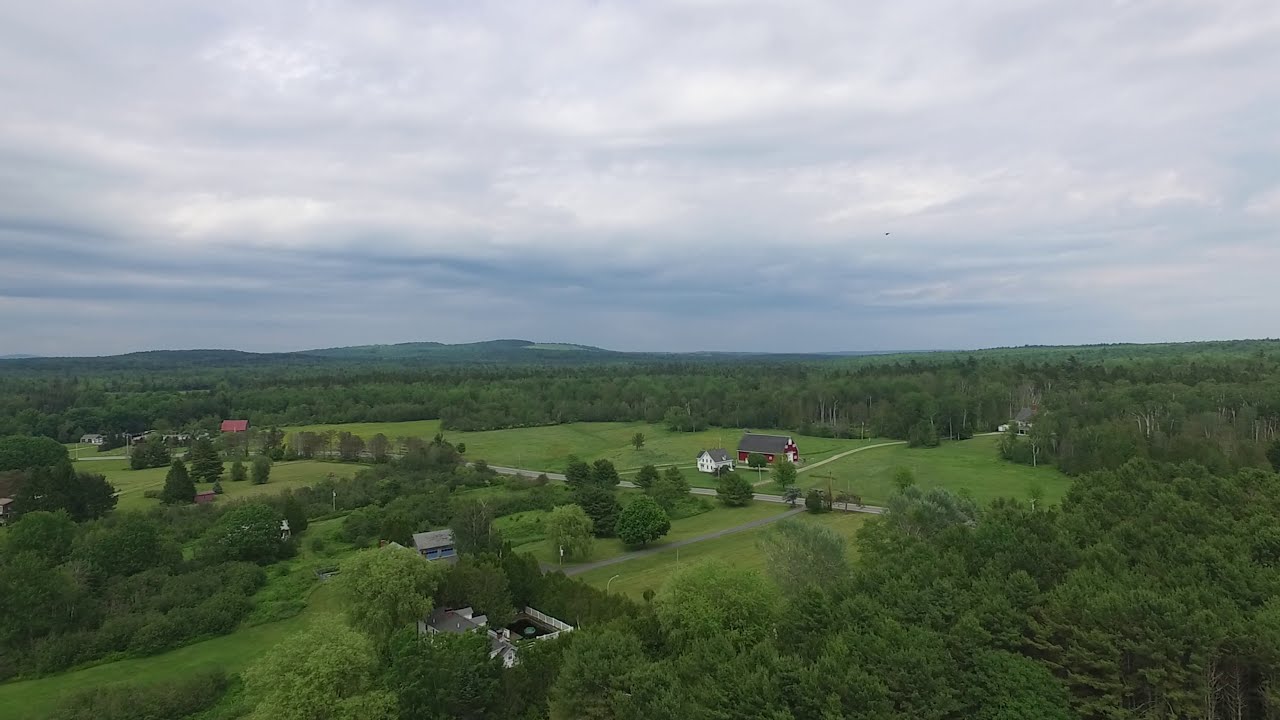The image is an aerial photograph capturing a rural landscape on a cloudy day. The sky, filled with white and gray clouds, dominates the top portion of the image, casting a natural, diffused light over the scene. Below the sky, a broad expanse of vibrant green grass and numerous trees covers the majority of the image. The landscape is dotted with several homes, including a noticeable red house and a white house near the center. To the left and in the bottom left corner of the image, additional homes are visible, blending into the tree cover. A road traverses the scene from the left, cutting through the center of the image and disappearing into a grove of trees on the right. The long driveways of the houses suggest they are set well back from the road, indicating spacious plots of land typical of rural areas. Surrounding the homes are fences, creating a patchwork effect in the greenery. The colors in the photograph are diverse, including green, red, white, blue, gray, and orange, contributing to a rich and detailed view of a serene countryside.